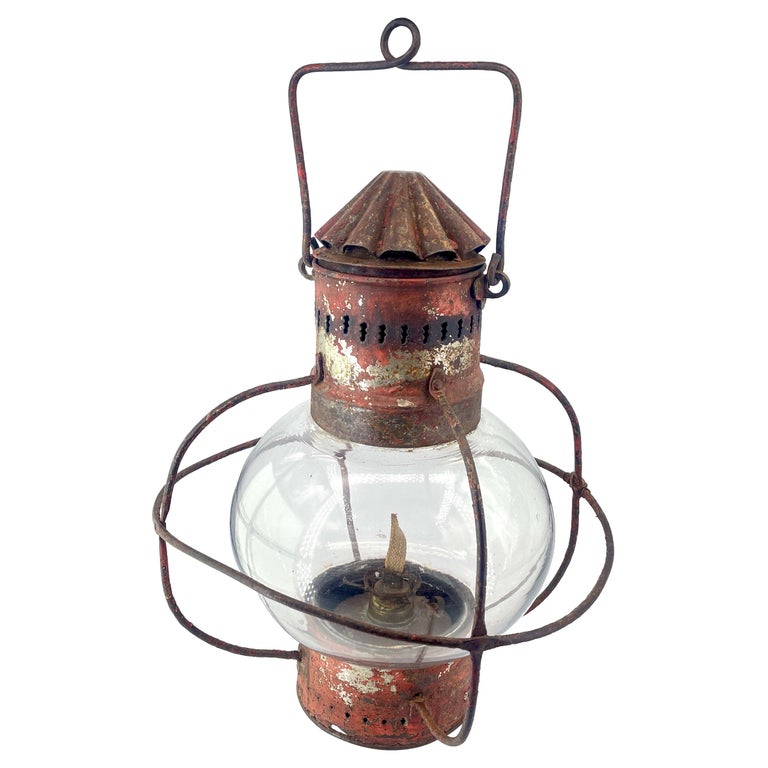The image features a heavily rusted, old-school lantern set against a completely white background. The lantern's metal, originally brown or possibly red, now displays a complex patina of gold, silver, dark red, black, and brown due to extensive rusting. The top of the lantern is detailed with an umbrella-like design and ventilation holes meant for releasing smoke and heat when the lantern is lit. A looped handle is affixed to the top, allowing the lantern to be carried or hung. The central section houses a glass bulb that encases a small wick, designed to be lit to illuminate dark spaces. Surrounding the glass bulb are protective metal bars or wires, shielded from impact. The lantern also features a dome-shaped bottom section, which likely serves to collect melted wax, enhancing its old-fashioned charm and utility.